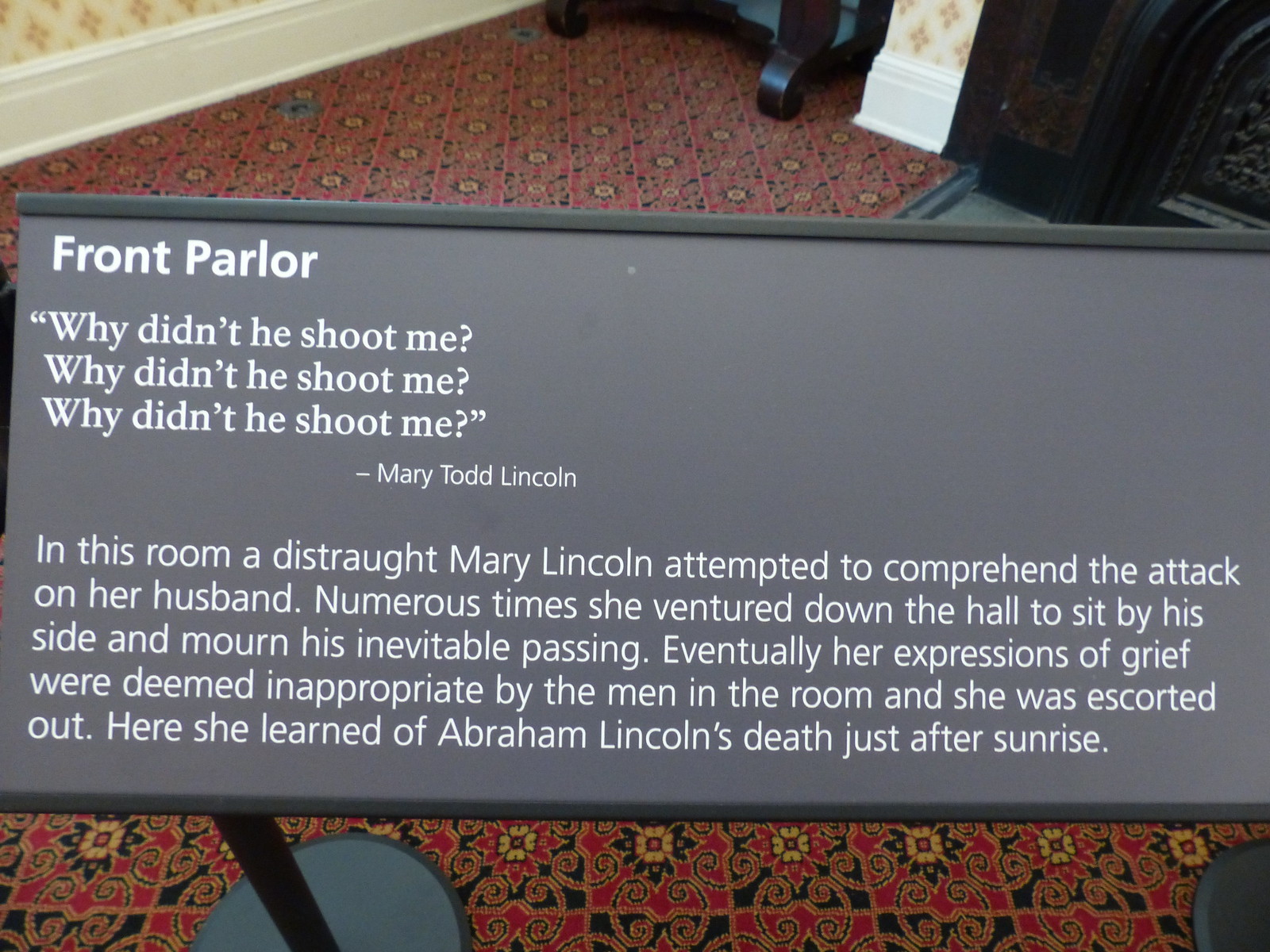The photograph showcases a museum exhibit placard, prominently displayed on two black pedestals and angled towards the viewer. This gray board features white text, dominated by the bold headline "Front Parlor." Below the heading is a haunting quote repeated thrice: “Why didn’t he shoot me? Why didn’t he shoot me? Why didn’t he shoot me?” attributed to Mary Todd Lincoln. The accompanying narrative describes Mary Lincoln's profound grief following the assassination of her husband, President Abraham Lincoln. The text recounts how she frequently left the parlor to sit by her husband's side in his final moments, only to be eventually removed by the men present for her emotional outbursts. It was here, just after sunrise, that Mary learned of his death. The placard is positioned over a striking dark red carpet adorned with floral medallion patterns. The scene hints at a historical room setting, partially visible with glimpses of baseboards and a potential doorway, adding depth and context to the emotional content of the display.